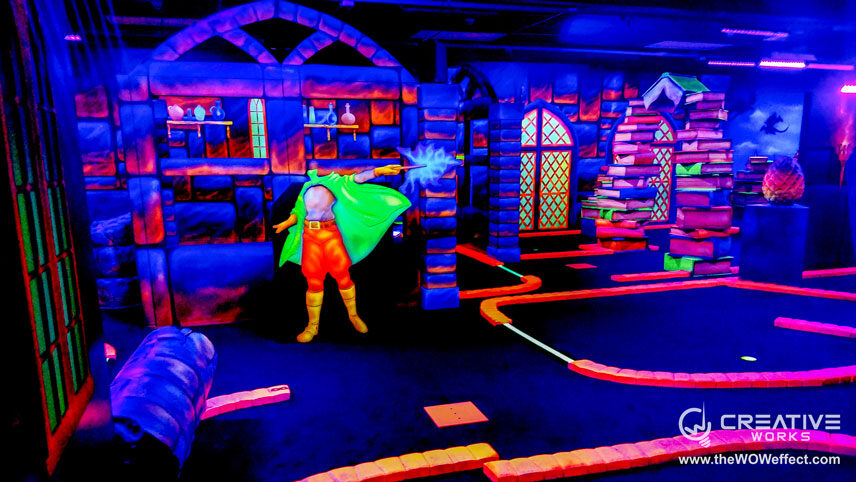This image, possibly an advertisement for a mini golf course by Creative Works (www.thewoweffect.com), is reminiscent of a video game interior or a fantastical children's play area bathed in vibrant neon electric hues. The scene is illuminated by ultraviolet lamps, resulting in striking fluorescent blues, greens, and oranges. The black matte floor is segmented by layers of vivid orange bricks, which create pathways throughout the space.

In the background, a mural features a wizard in bright fluorescent colors, wearing a green cape and holding a wand emitting blue light. The wizard, with a chest in ivory hues, orange pants, and yellow boots, stands against a backdrop that might be a wizard's tower or another fantastical structure. To the left, there appears to be a bar or scientific station with bottles and vials, emphasizing electric blue and red tones. 

A headless figure, possibly part of the mural or a stand-alone decoration, extends a wand, adding to the magical ambiance. A large stained glass window graces the center of the room, flanked by stacks of pink, blue, and purple books reaching from the floor to the ceiling. The area is vibrant, almost cathedral-like with round-shaped windows and pathways of electrifying colors, creating an enchanting and immersive environment.